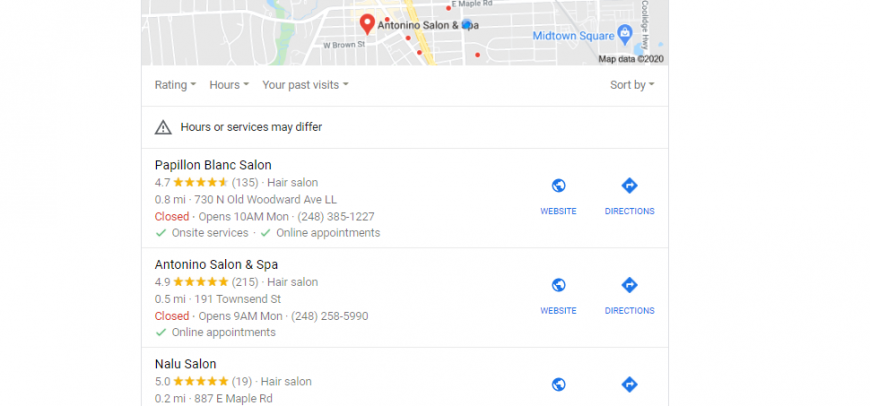The screenshot is from Google Maps, depicting a city map with streets shown in white against a gray background. At the top of the map portion, there is a red location marker labeled "Antonino Salon and Spa" in dark gray font. To the right, "Midtown Square" is indicated in blue font with a blue location marker beside it.

Below the map, the background turns white, and a top menu displays options: 'Ratings,' 'Hours,' 'Your past visits,' and 'Sort by' on the far right. Just beneath this menu, a note states "Hours or services may differ."

Three establishments are listed, all of which are salons. 

1. **Papillon Blanc Salon**:
   - Rating: 4.7 stars
   - Visual: Five gold stars, with the fifth star almost completely filled.
   - Options: 'Website' and 'Directions' in blue font on the right.

2. **Antonino Salon and Spa**:
   - Rating: 4.9 stars
   - Visual: Five fully filled gold stars.
   - Options: 'Website' and 'Directions' in blue font on the right.

3. **Nalu Salon**:
   - Rating: 5.0 stars
   - Visual: Five fully filled gold stars.